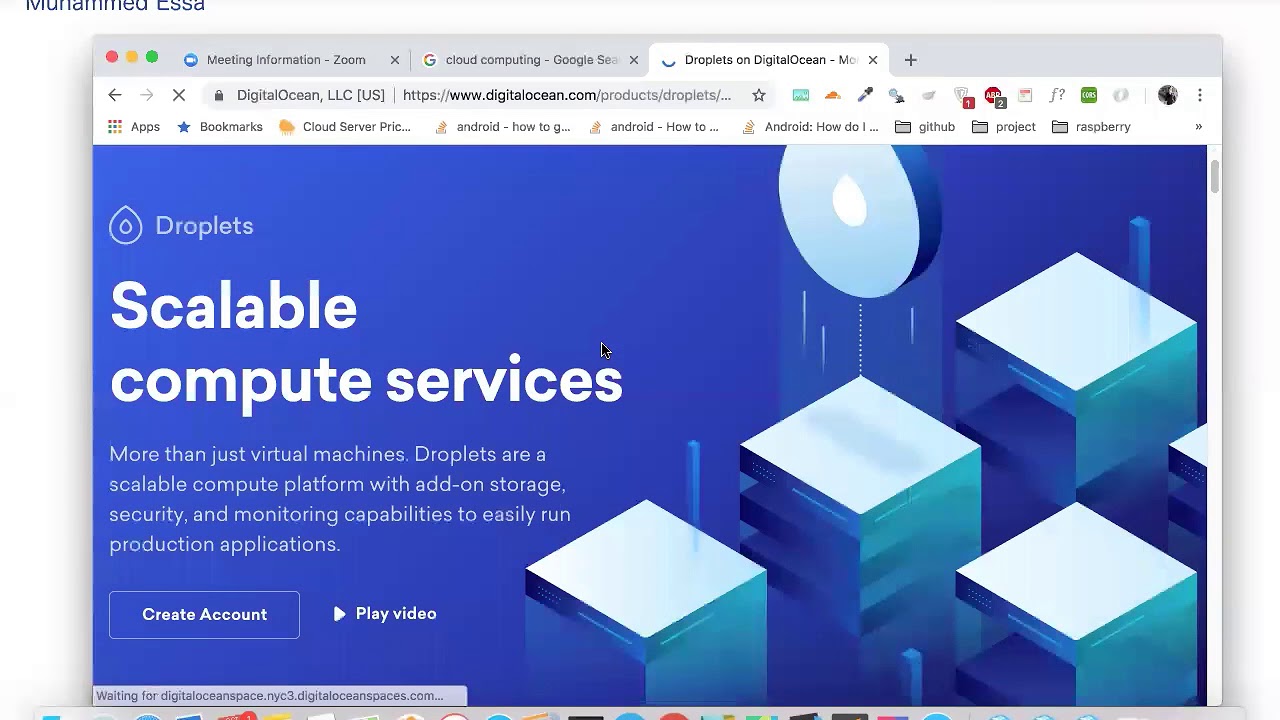The main page of the website prominently features the word "Droplets" in white font on the left-hand side, accompanied by a droplet-shaped logo. The primary background color is a rich blue. The focal image showcases an aerial view of angular blocks, resembling server racks, cascading diagonally from the top right corner to the center bottom. These blocks are not intricately detailed but convey the idea of scalable infrastructure. Below the "Droplets" heading, there is a tagline that reads "Scalable Compute Services," followed by a subtext emphasizing that the offerings extend beyond mere virtual machines.